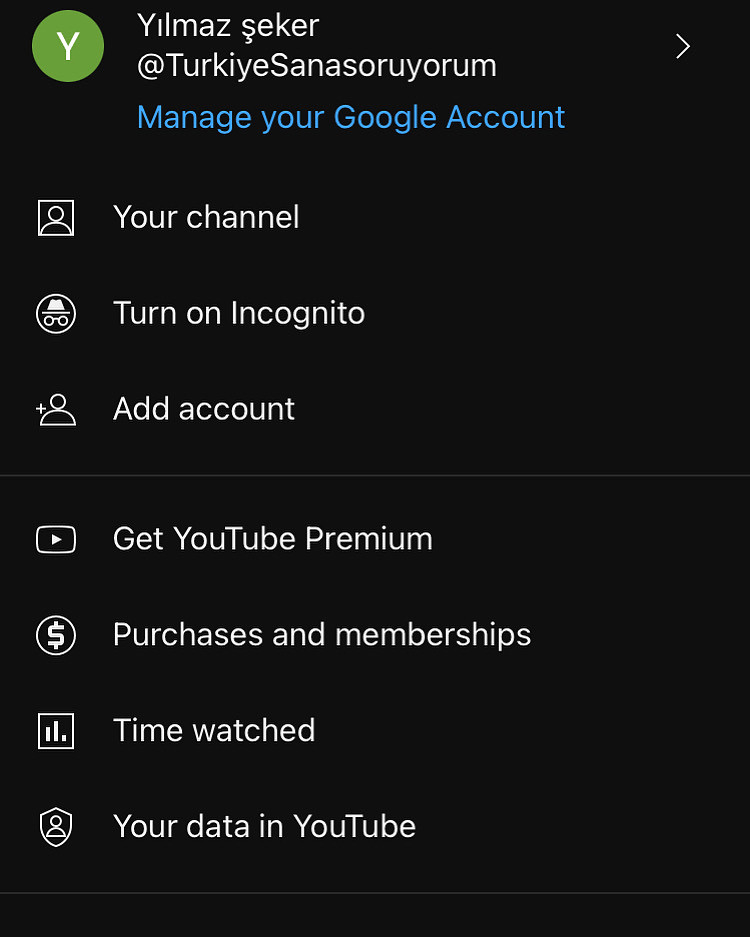The image features a flat, jet-black background devoid of texture and depth. Positioned vertically is a black rectangle. At the top left corner of this rectangle, there is a white circle enclosing a bold "Y". Adjacent to this, text in white reads, "YouTube Music". Beneath this text, in smaller white font, it states, "YouTube aSANTA SAORIUM." Directly below, in blue font, it prompts, "Manage Your Google Account."

In the top right corner, there's a familiar profile arrow icon, leading back. Underneath the "Manage Your Google Account" prompt, in white, is a small person icon accompanied by "Your Channel." Below this, within a circle, there's an icon of a hat and eyeglasses, labeled "Turn on Incognito." Next to it, a plus sign with a person icon tagged "Add Account" appears, separated by a thin line.

Further down, a play button icon appears with the offer "Get YouTube Premium." A dollar sign within a circle follows, with the label "Purchases and Memberships." The pattern continues with vertical bars arranged within a square symbolizing the "Time Watched" feature, and lastly, a badge icon reads, "Your Data in YouTube."

This meticulous alignment of icons and descriptions against the stark black background creates a visually ordered yet minimalist user interface depiction.